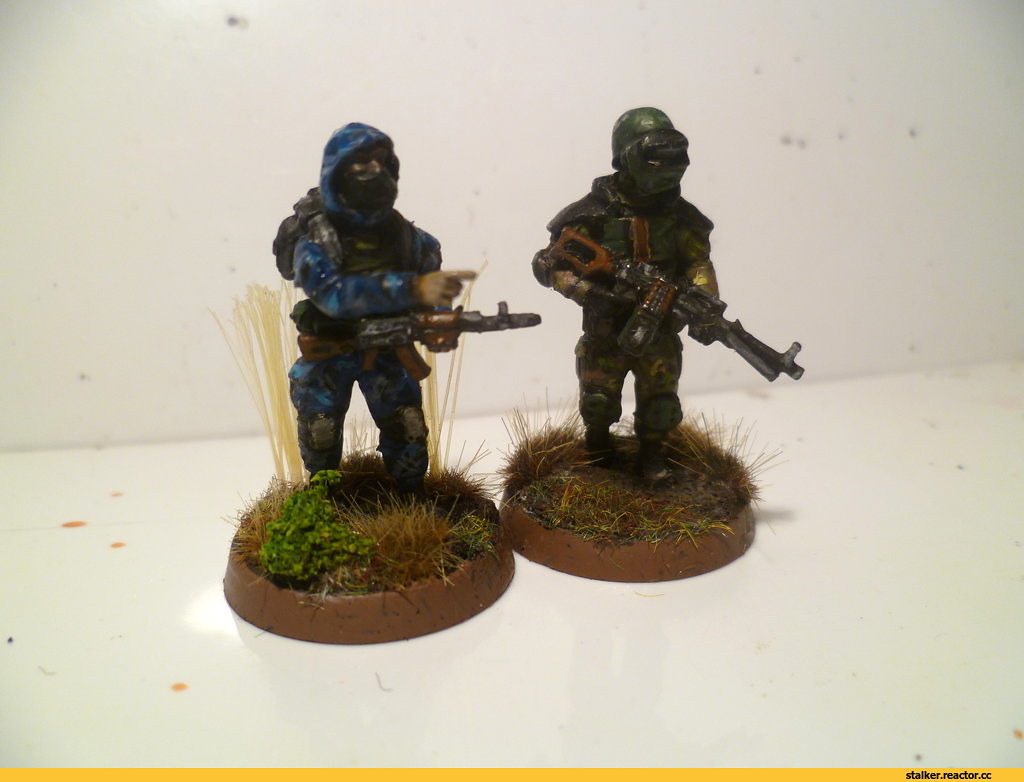The photograph captures two detailed military figurines standing on a white table with accidental red and black stains. The two toy soldiers, positioned at the center of the frame, stand on brown circular bases adorned with imitation grass and flowering plants. The backdrop is uniformly white with some black stains. The figurines give a strikingly lifelike military appearance, both adorned in camouflage uniforms. 

The soldier on the left is dressed in a blue camouflage uniform complete with boots, knee pads, a hood, and a face mask. He is holding an automatic rifle, positioned to his left, and appears to be pointing forward with his right hand. He's also carrying a backpack. This blue camouflage includes shades of blue, synchronizing with the overall military theme. 

The soldier on the right is in a green camouflage uniform, including a helmet and a face mask. He is armed with a larger gun, possibly a bazooka or a large automatic rifle, held in a right-handed configuration with the barrel facing left. Both figurines, around 3 inches tall, depict realistic details such as the varied shades of brown and green grass and plants at their feet, evoking scenes of a battlefield.